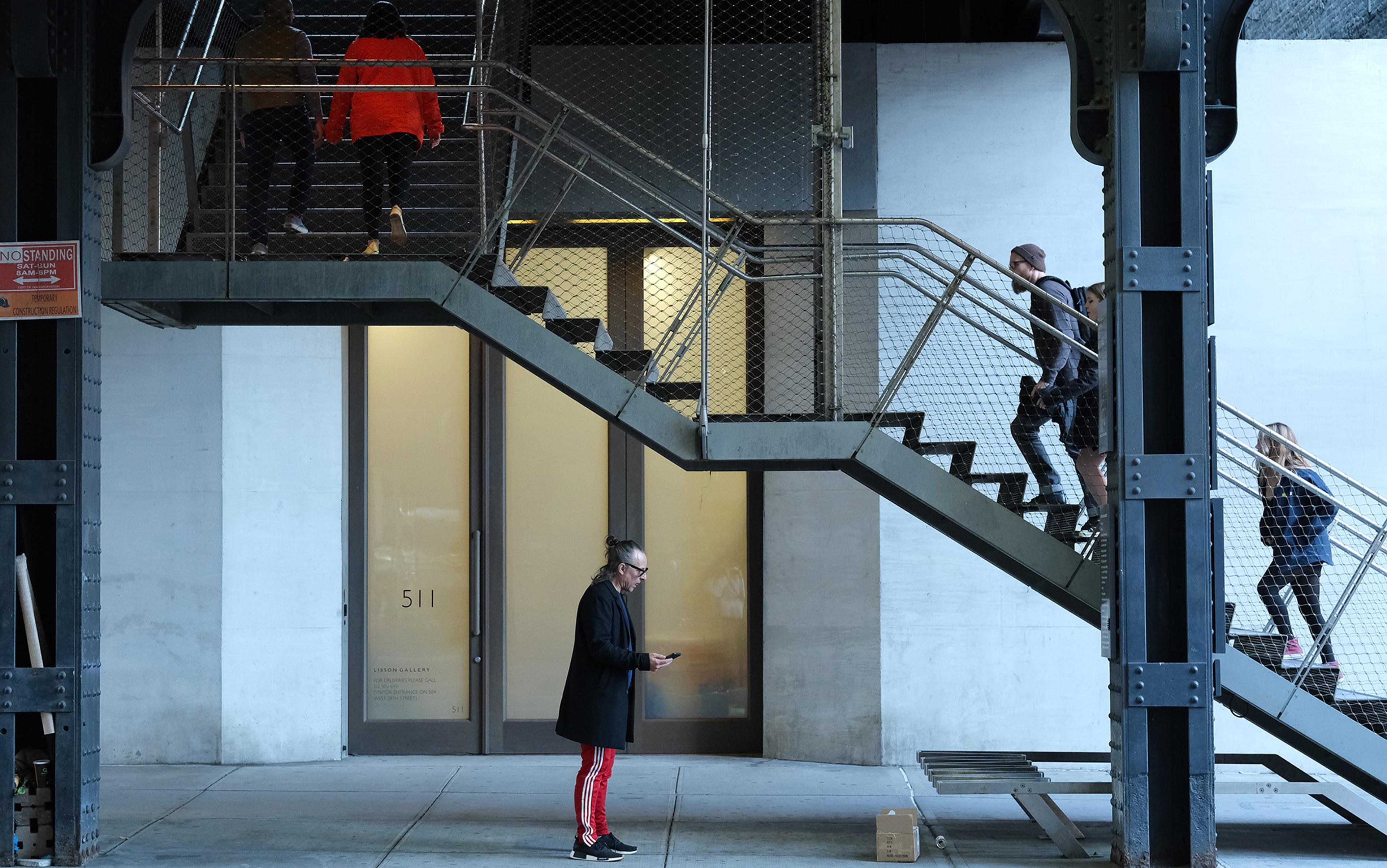In this grayscale photograph titled "Industrial Ascent," a scene of urban activity unfolds around a modern white and gray building numbered 511. Dominating the composition is a staircase weaving from the bottom right to the top left, bustling with human movement. Five individuals are navigating the stairwell, partially obscured by a steel girder: descending on the far right is a woman in a blue jacket, followed by a couple further up, the male in a gray jacket and glasses with short hair, and the female somewhat hidden behind a blue pillar. Ascending near the top left are a woman in a red jacket and a man in a leather coat. Below the stairwell, a bearded man in glasses stands engrossed in his phone. He's dressed in a contrasting ensemble of a black suit coat and red Adidas track pants, complemented by black shoes. This vivid portrayal highlights the layered dynamics of daily life within an urban setting, marked by a notable "No Standing" sign on the left, underscoring the ever-present motion.